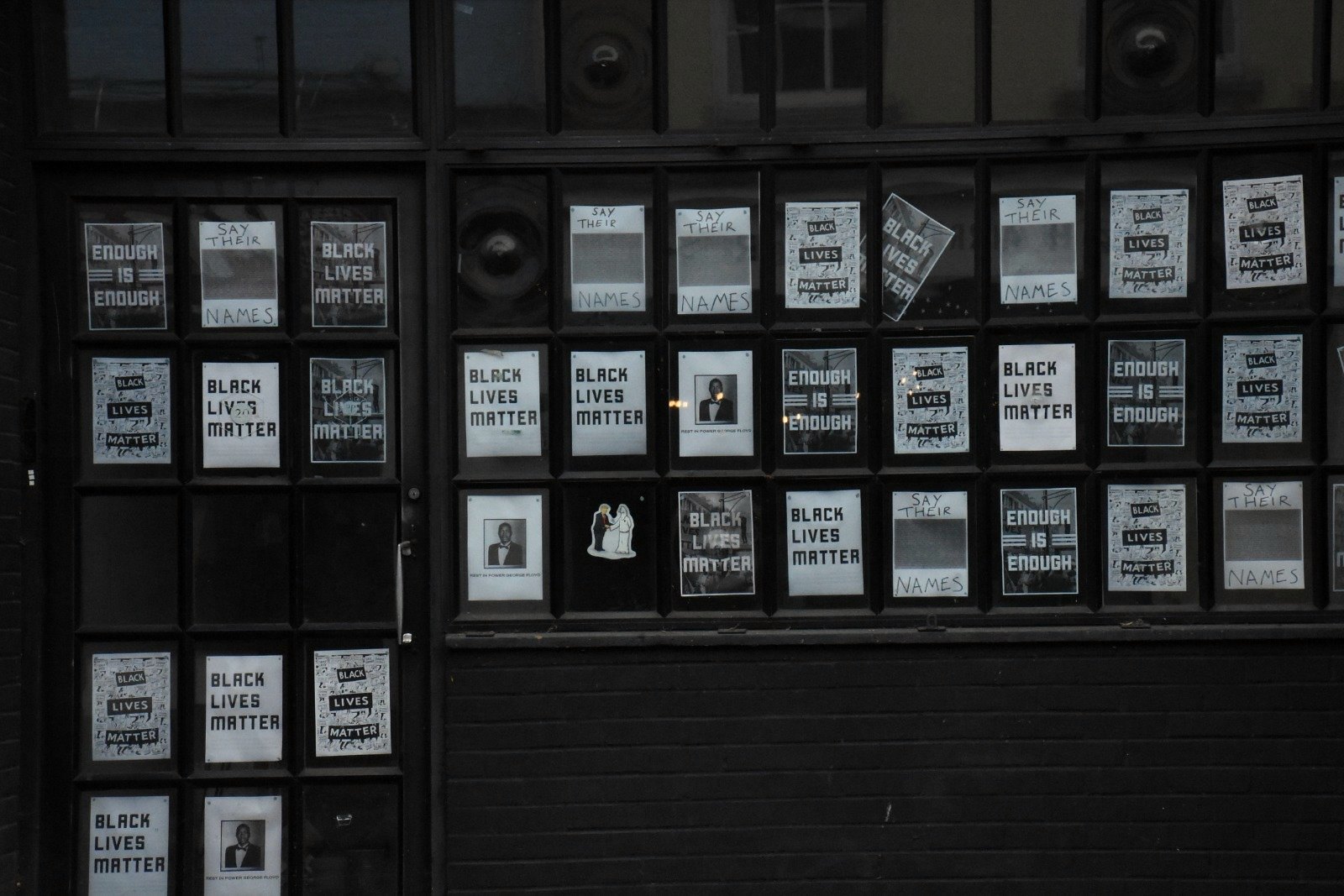The photograph depicts a dark, predominantly black wall structure that may be part of an outdoor display or a storefront. This structure is segmented into sections, with panels that appear to function as both windows and doors, adorned with numerous posters and book covers. The posters prominently feature slogans and titles related to the Black Lives Matter movement, including repeated messages like "Black Lives Matter," "Say Their Names," and "Enough is Enough." 

Three distinct types of panels can be seen: 

1. At the top are approximately 13 panels with book cover images, some showing titles like "Enough is Enough," "Say Their Names," and various iterations of "Black Lives Matter."
2. Beneath these are several more panels with similar themes and additional content, including a photograph of a man in a suit, suggesting a memorial or tribute. 
3. Lower panels reveal a black brick wall backdrop with three rows of posters, where titles like "Black Lives Matter" and "Enough is Enough" regularly reappear. There is also an illustration of a wedding couple.

Interspersed among the posters are what appear to be black circles resembling speaker covers, adding an audio-visual element to the display. The overall image is steeped in tones of black, giving it a monochromatic, somber feel, and is likely taken through a dark filter. The display case-like arrangement, combined with the reflective surfaces and a visible metallic door handle, suggests a sophisticated organization aimed at evoking contemplation and attention to the messages of racial justice and remembrance.